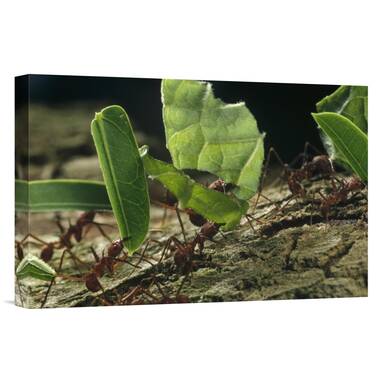This highly detailed, zoomed-in photograph captures the remarkable scene of red, leaf-cutting ants in action. The ants, characterized by their reddish-brown bodies, long legs, and prominent mandibles, are captured navigating a cracked, dry dirt landscape that slopes upward. The ants, arranged in almost regimented lines of two-by-two, demonstrate remarkable strength and coordination as they haul pieces of vibrant green leaves that are disproportionately large compared to their own bodies—some pieces even surpassing their size.

The image focuses sharply on the ants and the ground beneath them, while the background remains blurred, revealing hints of grass and a mixture of light brown and black hues, likely signifying a natural environment. The leaves, differing in size and shape, are held firmly in the ants' mandibles as they march collectively towards their colony, evoking a sense of organized labor commonly associated with tropical species such as those found in rainforests or the Amazon.

This photo, not a painting, showcases the ants in mid-motion, clearly on a mission to transport leaf segments either to their nest or another designated location. The vivid contrast between the green leaves and the dry, cracked earth beneath them emphasizes the industrious nature of these tiny yet formidable creatures. The sheer size of the leaf fragments in relation to the ants underscores the impressive physical capabilities and cooperative behavior of these worker ants.